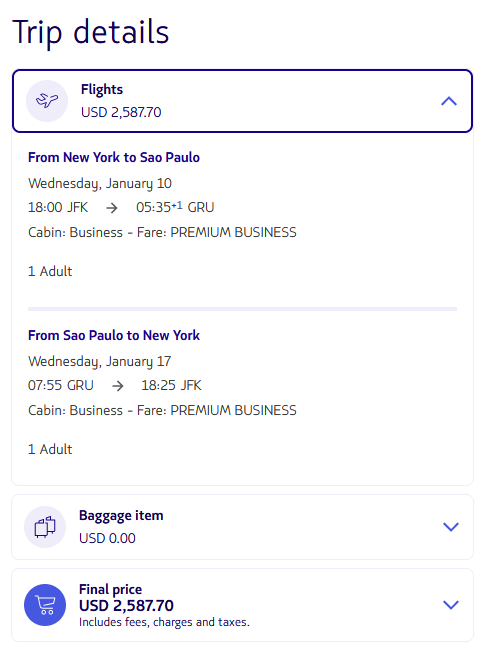This webpage predominantly features a white background. Prominently displayed in the top left corner, the text "Trip Details" is written in black font. Directly beneath this heading, there is a white box with a dark purple highlight. An icon of an airplane is positioned on the left side of this box. To the right of the icon, in black text, it reads "Flights," followed by the cost "USD $2,587.70" underneath. 

In dark purple text below the price, it states the route "From New York to Sao Paulo," along with the travel date "Wednesday, January 10th." Further details include "JFK $1800, GRU $535," specifying the departure and arrival airports. The seating class "Cabin Business" and fare type "Premium Business" are also mentioned, concluding with the passenger information "One Adult."

This description reflects a booking page for a flight being purchased, detailing the trip from New York to Sao Paulo with a total ticket price of $2,587.70.